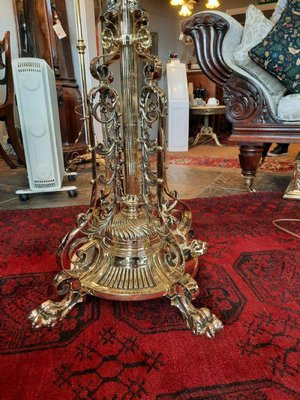In the center of the photo, positioned on a deep red carpet adorned with a snowflake pattern, there is an intricate, mystical-looking gold statue holding a sword. This antique piece, possibly the base of a bronze lamp with an ornate gothic design, is surrounded by an assortment of old-fashioned items indicative of a living room setting. In the background, various objects can be seen, including a chair, a couch, a teapot, and push-type radiators on wheels. The overall aesthetic is antique and somewhat mysterious, capturing an indoor scene with rich, warm colors like dark red, gold, and brown, though the lighting and time of day are indeterminable.